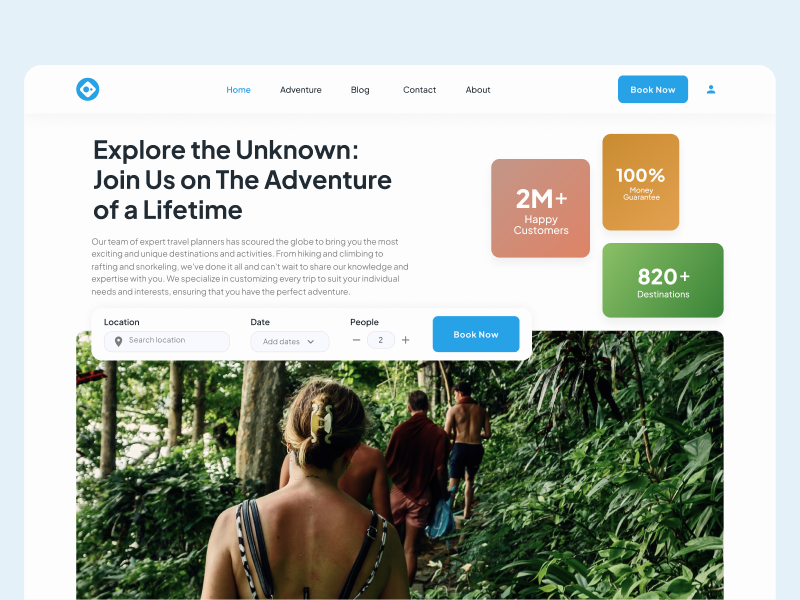Screenshot of a travel website featuring a clean and user-friendly design. **Layout**: 

- **Central Element**: The focus is a prominent white square at the center, occupying the majority of the screen.
- **Top Navigation**: 
  - **Logo**: Positioned at the top left, a blue circle enclosing a white diamond and a smaller blue circle.
  - **Menu Options**: To the right of the logo, menu items are listed in black text with "Home" highlighted in blue. Options include Home, Adventure, Blog, Contact, and About.
  - **Top Right Features**: A "Book Now" button with white text on a blue, curved-edge box, alongside a blue profile icon.

**Content**:

- **Main Heading**: Below the navigation, on a grayish background, large black text reads, "Explore the Unknown. Join us on the adventure of a lifetime."
- **Descriptive Paragraph**: Positioned underneath the main heading in smaller text.
- **Statistics and Guarantees**:
  - **Box 1** (Soft Red, Curved Edges): "2M+ Happy Customers" in white text.
  - **Box 2** (Orange Vertical Rectangle): "100% Money Guarantee" in white text.
  - **Box 3** (Green Horizontal Rectangle): "820+ Destinations" in white text.

**Main Image and Search**:

- **Image**: A large image at the bottom depicting four people hiking through a jungle, viewed from behind. The lead hiker, a woman with blonde hair tied up in a clip and wearing a swimsuit, is followed by three men; two are shirtless, and the third has a red towel over his shoulder.
- **Search Box**: Located below the image, featuring adjustable fields for Location, Date, and People. A prominent blue "Book Now" button completes the form.

This detailed caption encapsulates the website's adventurous spirit and user-oriented layout, designed to engage potential travelers.